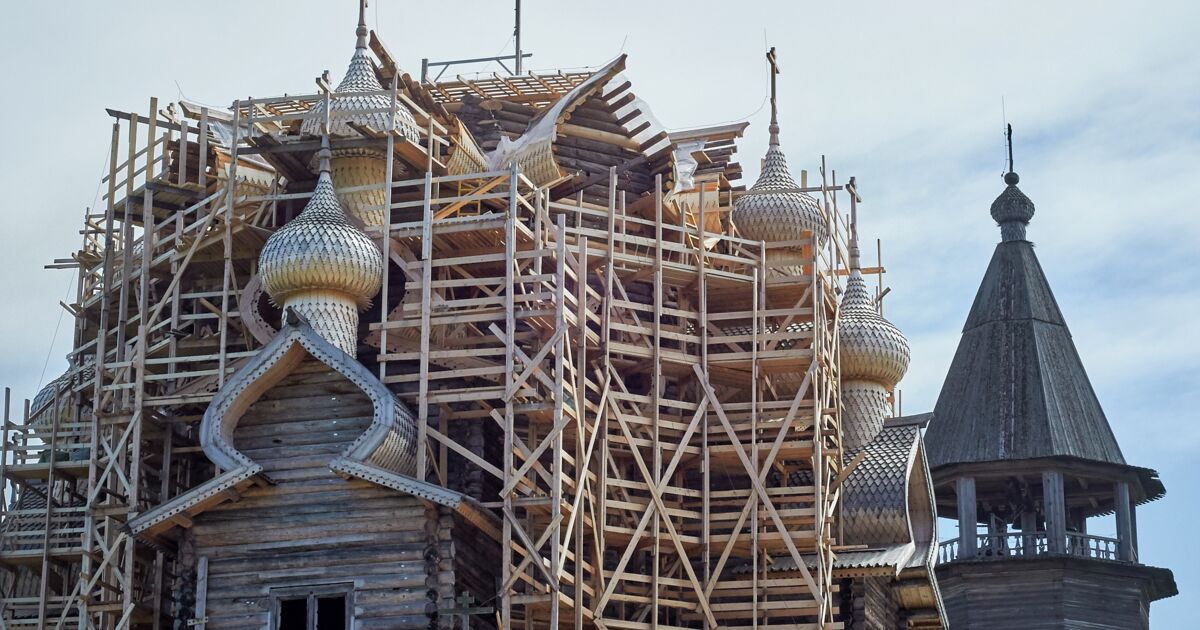This colored photograph captures an impressive cathedral undergoing renovation. The prominent feature is the extensive wooden scaffolding covering most of the building's facade, constructed from multiple small 2x4s, creating a complex web reminiscent of matchsticks. The cathedral itself is distinguished by several golden towers, each crowned with a cross, contrasting with the weathered wood of the building. These golden towers exhibit a spiky, crown-like design, with metal panels that gleam in the light. To the right of the primary structure stands another tower, made entirely of unfinished wood, ascending to a pointed cone shape. This wooden tower includes an accessible area beneath its roof, supported by wooden posts with a railing walkway visible. The aged and rustic appearance of the cathedral, combined with the intricate scaffolding and varied tower designs, reveal the historic and architectural richness of the building.